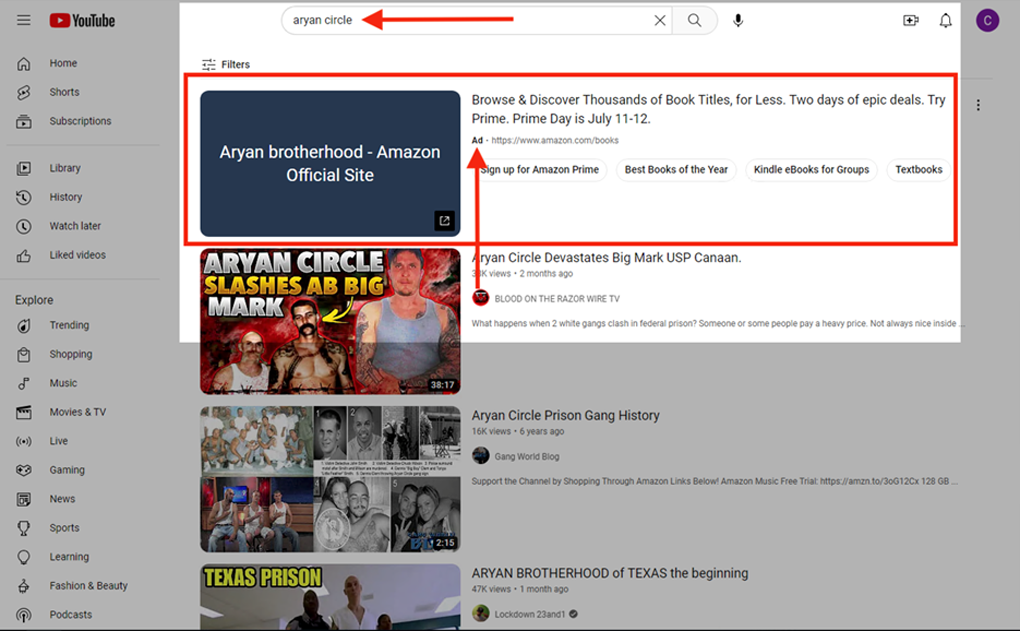The image depicts the YouTube home screen with several distinctive elements. Starting from the left and moving in about 2 inches, then halfway down the screen, and a further inch from the right, the background is a light grayish color.

In the top-left corner, there are three black horizontal lines, symbolizing the menu. Next to it is the red YouTube play button, followed by bolded black text that reads "YouTube." Beneath this, there are various navigation icons listed vertically on the left. Each icon is accompanied by its corresponding name on the right, starting with:

- Home
- Shorts
- Subscriptions

A horizontal line follows these icons, with additional categories below, including:

- Library
- History
- Watch Later
- Liked Videos

Another horizontal line separates these categories from more listed icons, under the heading "Explore," detailing:

- Trending
- Shopping
- Music
- Movies & TV
- Live
- Gaming
- News
- Sports
- Learning
- Fashion & Beauty
- Podcast

At the very top of the screen, where the gray area turns white, there is a search bar labeled "Arian Circle," marked by a prominent red arrow pointing to it. Further to the right of the search bar, there’s an "X" button, followed by the search icon, voice search icon, and a bell icon. In the top-right corner, a small purple circle with a "C" inside it appears against a blue background.

Below the search bar, there is a "Filters" button positioned slightly to the left. A red-bordered rectangle spans from left to right, containing a blue box with the text "Arian Brotherhood-Amazon," followed by the title "Official site" and additional information on the right. Below this, an image with the text "Arian Circle slashes a big mark" accompanied by further information to the right is visible, followed by two more similar entries underneath.